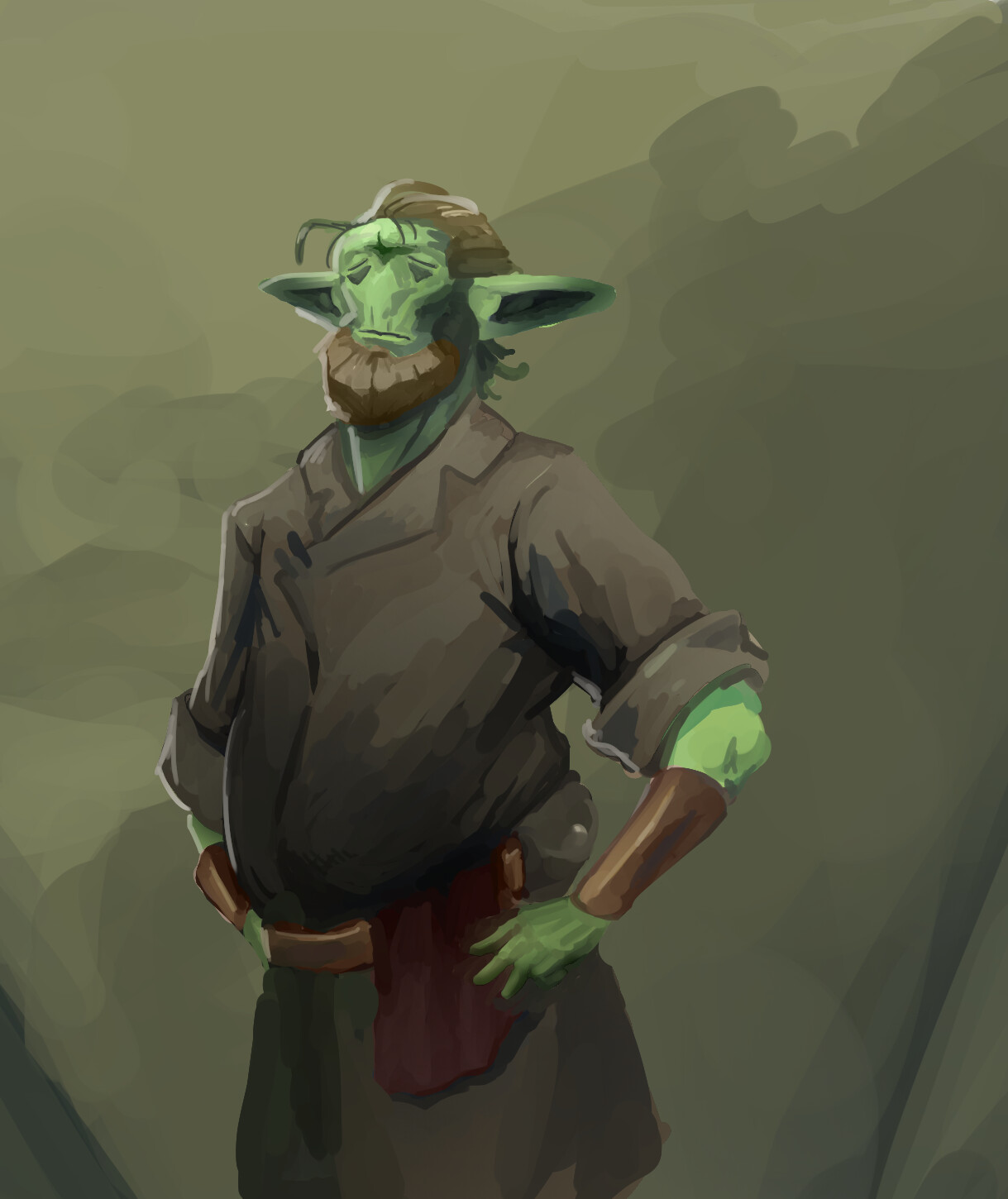This artwork is a detailed watercolor painting featuring a green orc with a notably large, pronounced belly, akin to Santa Claus. The orc has pointy, long green ears and a saturnine expression characterized by downward-facing triangle eyes, an absent nose, and a simple-line mouth. He sports a bushy, brown beard and brown hair, somewhat reminiscent of Abraham Lincoln's iconic look. He is dressed in a dark brown, heavy coat with a brown belt around his waist, from which a red washcloth dangles. His outfit includes brown arm guards at the wrists. The watercolor background is an abstract mix of light brown, dark brown, and gray hues without any defined features, lending a modern art vibe to the piece. The overall lack of detail in the orc's facial features contrasts with the colorful and indistinct backdrop of muddy browns and grays.